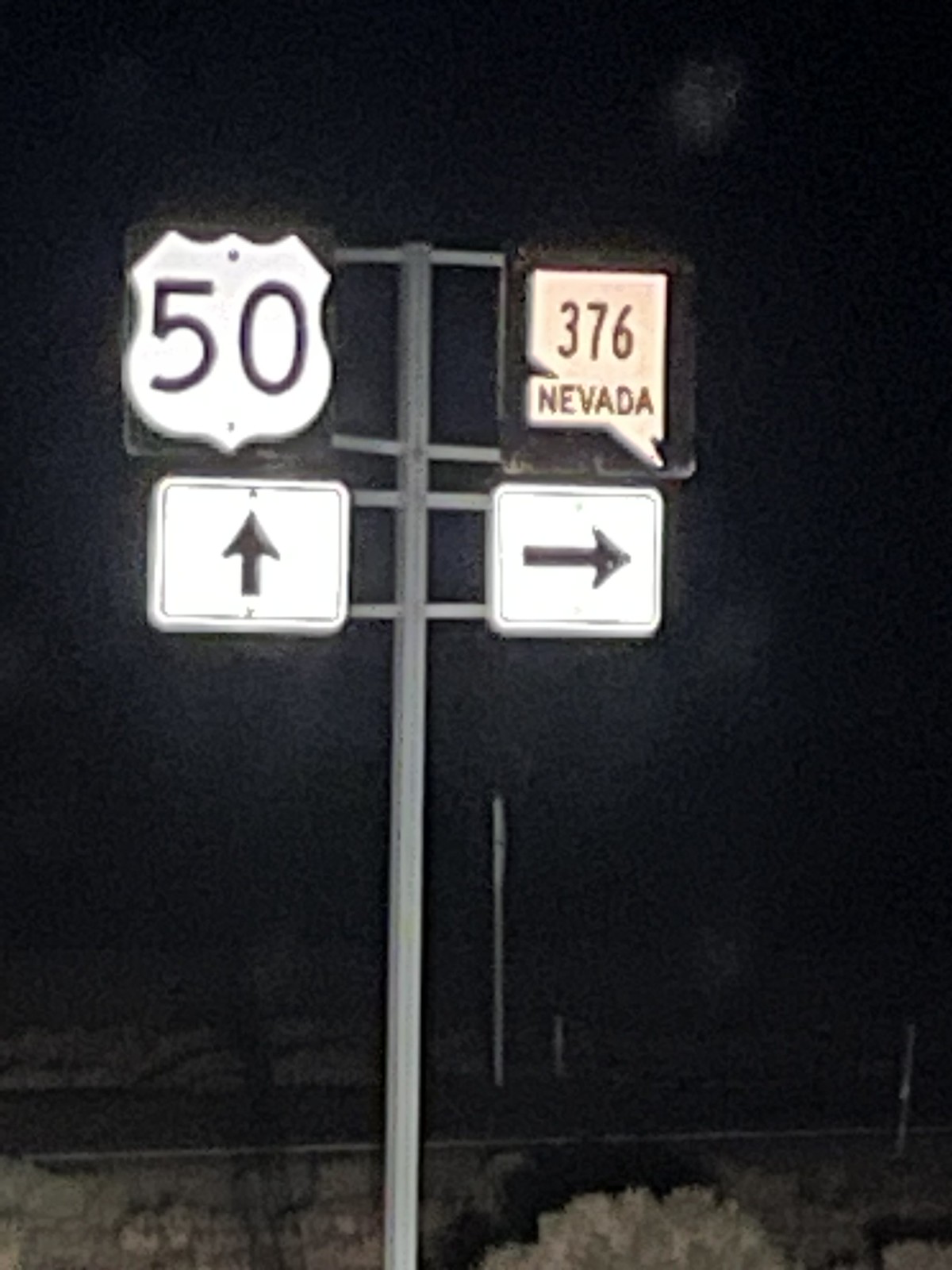This is a black and white photograph of a street sign taken at night. The image is blurry and out-of-focus, giving it a low-quality appearance. The background is starkly black, creating a high contrast with the illuminated signs. A single metal pole supports four signs arranged in a two-by-two grid. 

On the upper left is an interstate shield with the number 50, indicating it's part of Interstate 50. Below this, a small white square sign with a black arrow points straight up, suggesting forward movement. On the upper right, there's a sign in the shape of the state of Nevada; it features the number 376 in black, with "Nevada" written underneath. Below the Nevada-shaped sign is another square white sign with a black arrow pointing to the right, indicating a right turn. 

The bottom of the image is somewhat ambiguous due to the darkness, but it looks like there could be a small wall or sidewalk with some scrubby vegetation on either side. The overall composition focuses heavily on the gray pole and the distinct signs against the nighttime backdrop.